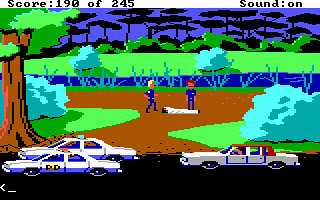In this image, a still from an 8-bit style video game is depicted. In the foreground, there is a black road occupying roughly a quarter of the screen. On this road, three cars are driving to the left: two police cars and one civilian car. The police cars, which appear to be unoccupied, are white with blue streaks along the bottom. The civilian car is entirely white with a brown top section, and it has a driver inside.

To the left of the road, a pathway leads to a park scene. In this park, two police officers stand over a body covered by a white tarp. The officer on the left has blonde hair, while the one on the right has brown hair, indicating they are investigating a potential crime scene, likely a murder. In the background, a river and trees are visible, adding depth to the scene.

In the upper left corner of the screen, the score "192.45" is displayed, and in the upper right corner, the text "sound on" is shown, indicating game settings.